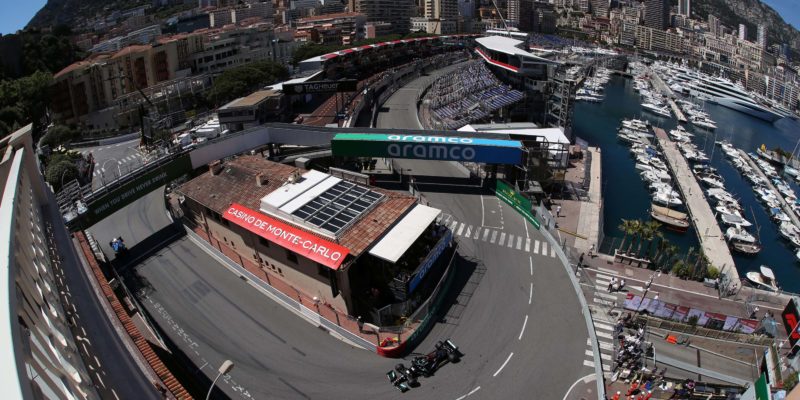Aerial fisheye photograph of a bustling Monte Carlo scene on a sunny day. In the foreground, the curved, distorted edges of the lens capture a detailed view of a large, brown building prominently displaying the name "Casino de Monte Carlo." This structure is encircled by a Formula One racetrack, which makes a sharp S-curve through the city and is marked by the green and blue Aramco signage. Several elongated race cars navigate the turns, while barriers lining the track hold back spectators. To the right, a bustling marina is filled with various boats and giant yachts, all neatly docked. On the left side of the image, a stone railing or bridge fence is partially visible, suggesting the height and elevated vantage point of the photograph. The background reveals towering city skyscrapers built into the base of a mountain, offering a striking contrast between the modern architecture and natural elements of the scene.